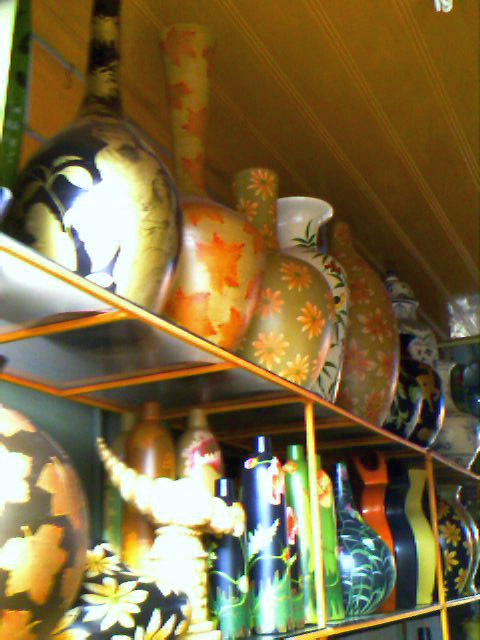The image depicts an exquisite display of pottery carefully arranged on a two-tiered shelf. The shelves appear to be made of glass with golden metal supports, adding a touch of elegance to the overall presentation. The ceiling above is a beadboard stained in rich brown hues, featuring line designs indented in an orangey-tan shade, giving a warm, artistic touch to the space.

On the top shelf, closest to the ceiling, stands an array of tall pottery pieces, masterfully decorated in a palette of tan, orange, white, and blue. The designs predominantly feature intricate floral and leaf motifs, creating a vibrant and nature-inspired collection. The varied shapes and sizes of these pieces demonstrate the artisan's skill and creativity.

The second shelf, not quite as in focus, showcases smaller and somewhat more slender pottery items with diverse forms, including some that resemble narrow water bottles. These pieces are adorned in shades of green, dark blue, orange, and yellow, boasting a mix of floral designs and striking stripes. Despite the soft focus, the artistry and the detailed decorations on these pots are evident, suggesting a vibrant and cohesive aesthetic that unites the entire display.

Overall, the photograph captures a beautiful, meticulously arranged collection of pottery, blending artistry and functionality, likely in a small shop or studio setting where these unique pieces are exhibited for admiration and purchase.